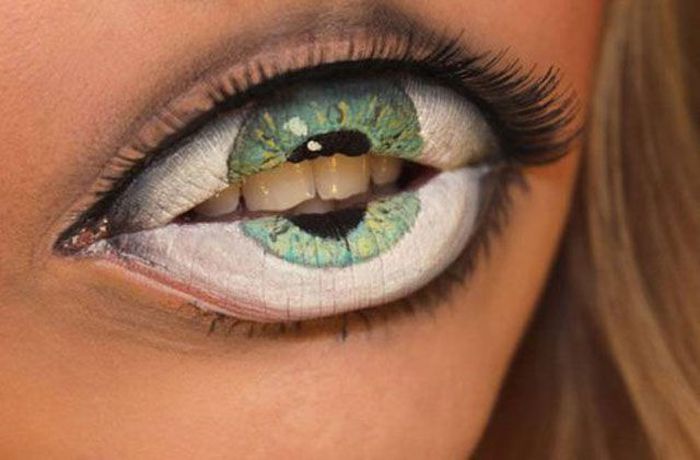This intriguing image showcases a striking visual illusion of a mouth expertly painted and styled to resemble a grotesque eyeball. The lips are meticulously covered with white paint, creating the sclera, while shades of blue and green form the iris, and a vivid black dot represents the pupil. Unexpectedly, the mouth opens to reveal a set of teeth, appearing as if they are emerging from the pupil itself. Delicate, finely drawn eyelashes frame the top and bottom of the 'eye,' with longer lashes predominantly sweeping outwards on the right side and shorter ones tapering off to the left. The same pattern is mirrored along the bottom edge of the 'eye,' enhancing the illusion. In the background, strands of dirty blonde hair subtly peek through, suggesting the location on the face aligning where the lips naturally are. This close-up shot centers on the lips, yet at first glance, it convincingly mimics an unsettling eye with teeth. The level of detail in the painting and illusion artistry is truly remarkable.